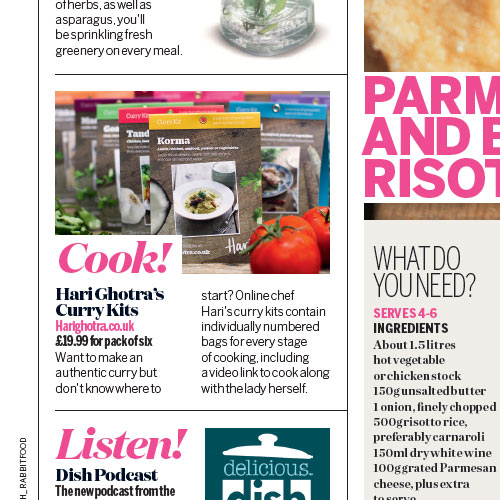The image features a clean, well-laid-out screenshot of a food or cooking page, divided into four distinct sections by a black line. The layout includes three columns on the left side and one on the right, though the top, bottom, and right sections are only partially visible. The middle column on the left is fully in frame and displays a detailed image of spice packets. The first packet prominently shows the label "Korma," suggesting it is for an Indian Chicken Korma. To the bottom right of the packet, there are tomatoes, and below the product, the word "Cook!" is written in pink lettering. Just underneath that, the text reads "Horigotra's Curry Kits," indicating a brand or product line. To the right, partially visible, there appears to be a recipe section. Some text related to a farm and possibly a zoo is cut off, but it suggests an additional context or theme for the content.